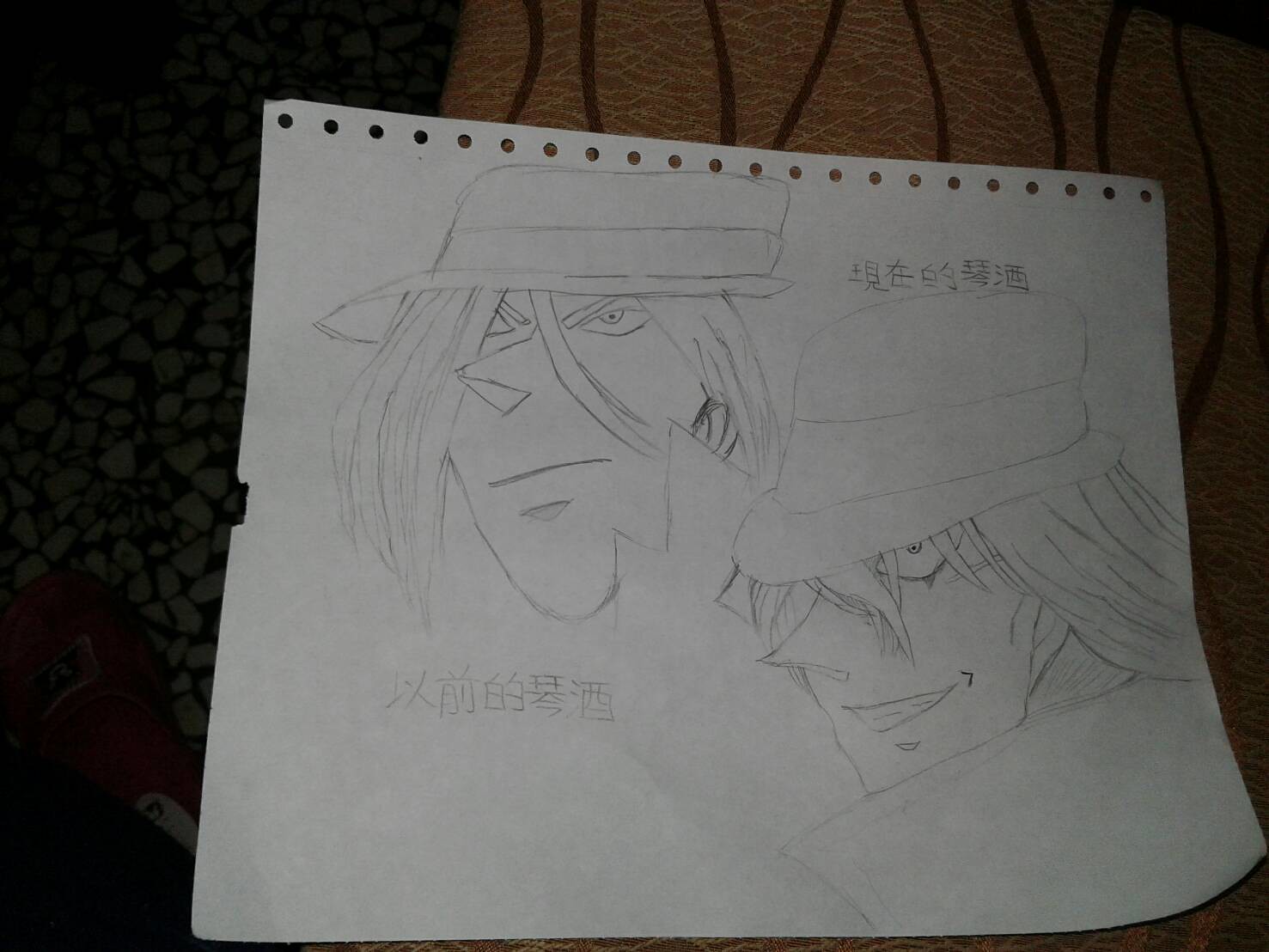This is a photograph displaying a pencil sketch on a piece of paper, which appears horizontally larger than it is vertically. The dark, textured backdrop in shades of brown gives the impression the paper might be resting on a pillow. The top edge of the paper bears perforations reminiscent of old dot matrix printer paper, adding a vintage touch. The sketch itself is rendered in an anime style, featuring two male faces. The character in the upper left has long hair draping down to his chin, obscuring his right eye, accompanied by a somewhat triangular nose. The character on the right exudes a sinister aura, reminiscent of "A Clockwork Orange" with his fedora tilted over the bridge of his nose and a malevolent grin. Additional Chinese lettering decorates the space above the right figure and below the left face. Notably, there is a small tear on the left edge of the paper, adding to the sketch's worn appearance.